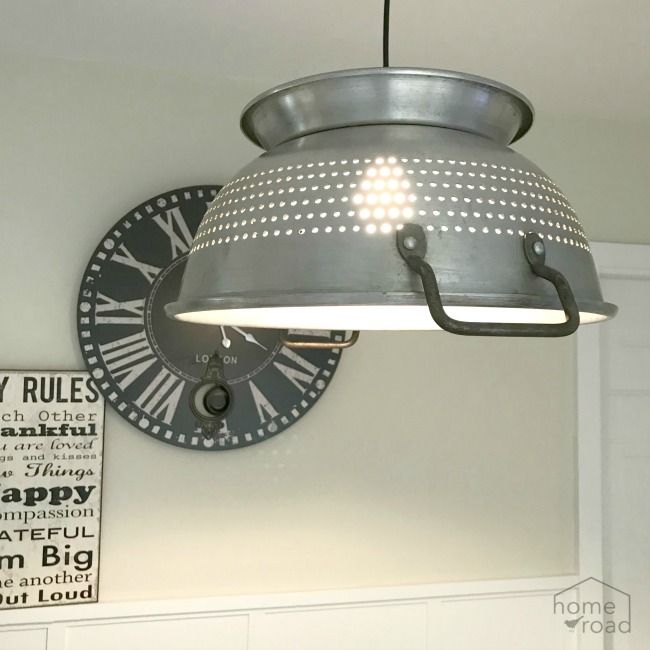This photograph captures a creatively repurposed metal colander transformed into a hanging lampshade, dominating the upper half of the image. The colander, made of silver metal, is suspended upside down from a black wire and emanates bright, white light from the exposed bulb within. It features a band of six rows of small holes around its middle and dark, rounded handles on either side. Behind it, a part of a white wall is visible, along with the edge of a white door on the right side of the photograph.

To the left, there's a round, black clock adorned with Roman numerals. Additionally, a partially readable black-and-white sign, similar to those found in home goods stores, displays words such as "rules," "thankful," "are loved," "happy," "compassion," "grateful," "big," "another," and "out loud." The light gray, cream-colored wall serves as the backdrop, and a watermark reading "Home Road" is located in the lower right corner of the image. Together, these elements suggest a homey, rustic aesthetic, possibly in a kitchen or dining area.